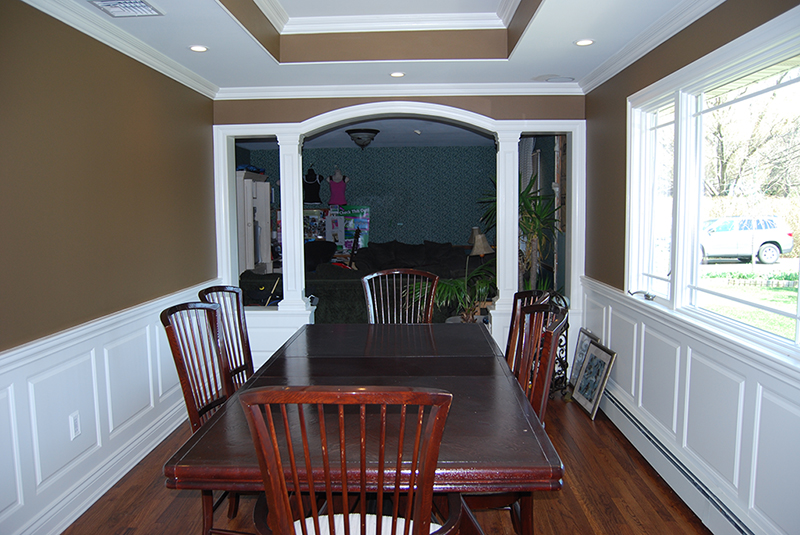This is a detailed description of a dining room, possibly just moved into or intended for real estate listing, though not fully staged. The room prominently features a long, rectangular cherry wood dining table surrounded by six chairs—two on each side and one at each end. The space is characterized by its contrasting wall colors: the upper portions are painted a warm brown, while the lower sections, adorned with paneled, white square designs, give a balanced, elegant look. The ceiling has a recessed, white center with brown edges, suggesting possible architectural detailing or a skylight.

The dining room has rich, dark hardwood floors that complement the table's reddish-brown hues. There are notable details such as a large window with white wood molding on the right side and an arched doorway with bright white framework at the far end, leading into a living area. This adjacent room appears cozy, with a couch against a bluish wallpapered wall and lamps adding ambient light. Several pictures are propped against one wall, indicating they may either need to be hung up or are awaiting packing, adding to the sense that the space is in transition.